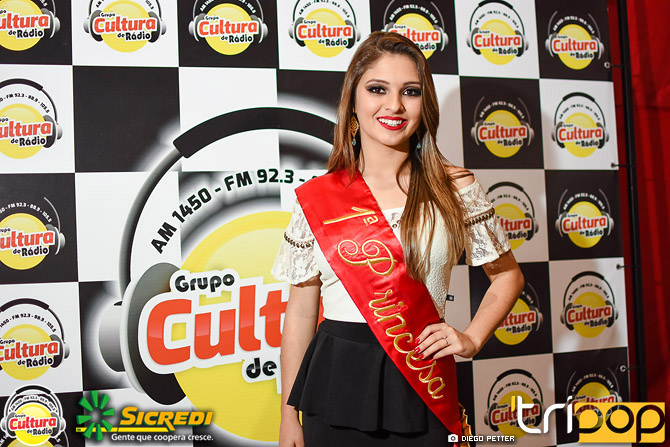This color photograph captures a young woman standing proudly, her long, light brown hair cascading over her shoulders. Dressed in an off-the-shoulder white top and a black skirt, she exudes confidence. Adorning her outfit is a prominent red sash with gold print that reads "One Princess." Her striking appearance is further accentuated by her red lipstick, dangling earrings, and nails painted a matching red. She poses with one hand on her hip.

Behind her is a horizontally rectangular backdrop, likely supported by black metal rods. This backdrop features a black and white checkered pattern, with each square containing a yellow circle emblazoned with red-lettered text that reads "Kaltura Radio." Larger text on the backdrop displays the radio station's frequencies: AM 1450 and FM 92.3. Additionally, the bottom right corner of the image bears the text "Tri-Pop" in white, set against the backdrop. This photograph likely commemorates her victory in a contest, underscored by the celebratory setting and the detailed promotional imagery behind her.